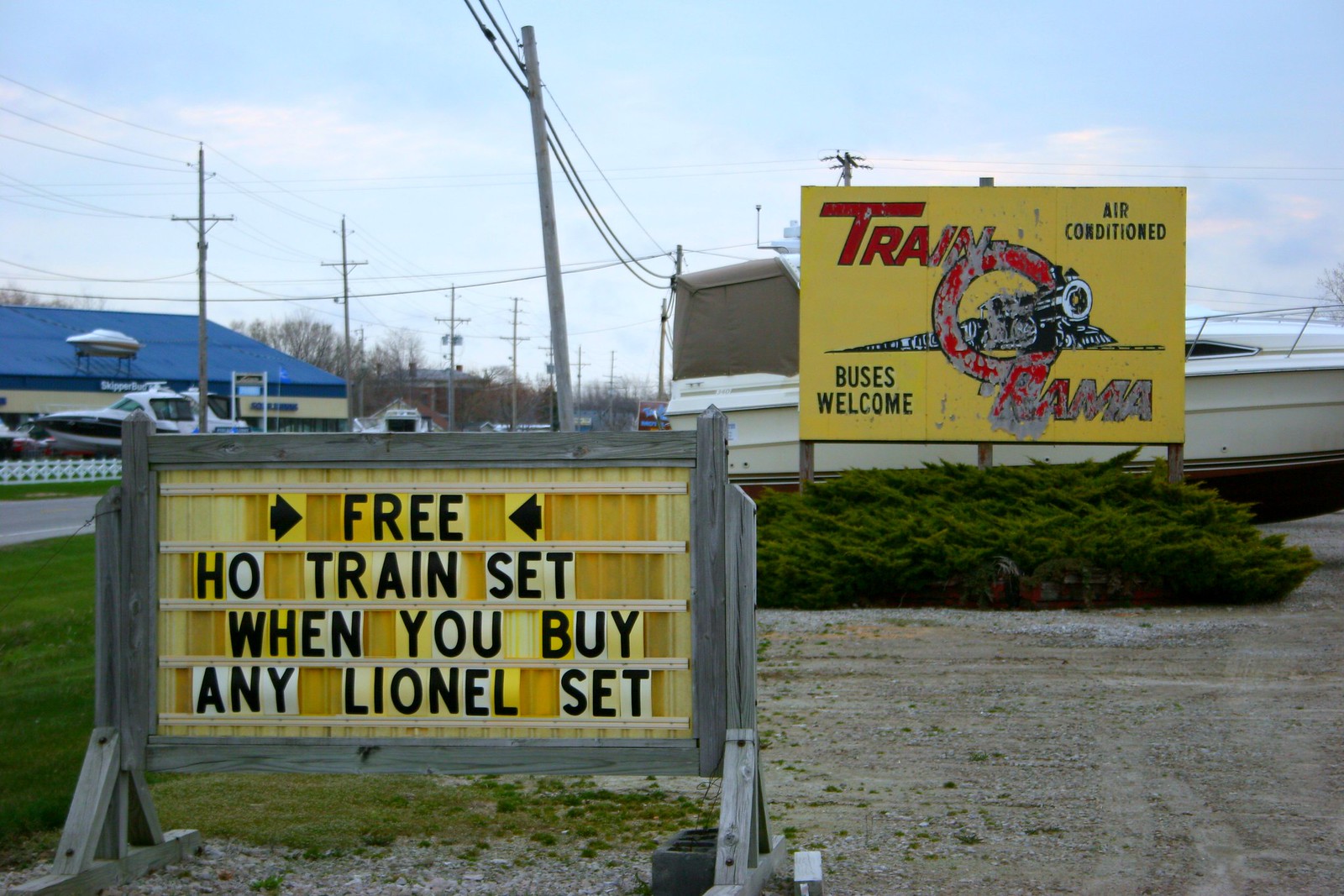The photo captures an outdoor scene in what appears to be a shipyard or train yard, set against a backdrop of distant trees and a street lined with electricity poles and wires. A blue-roofed building and a boat on a trailer can be seen in the background. On the right, partially obscured by a weathered yellow sign with red and black text, is a large white and blue boat. The yellow sign reads "Train-O-Rama" in red text, accompanied by a picture of a black train on its mantle, with additional black text stating "Air Conditioned" and "Buses Welcome." In the gravel parking lot foreground, a green bush grows out of the ground, and there is an interchangeable letter sign with a yellow background and wooden frame. The black letters on this sign read, "FREE HO TRAIN SET WHEN YOU BUY ANY LIONEL SET." Additionally, there is a wooden customizable sign on the bottom left with arrows pointing to the word "FREE" and stating "Ho Train Set When you buy any Lionel set." The scene also features boats parked across the street in adjacent lots.